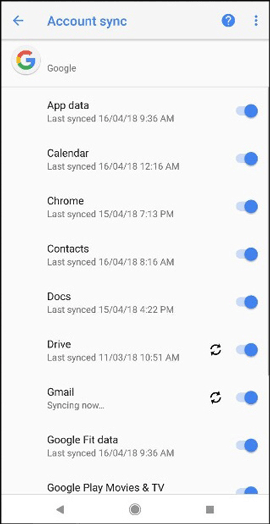This is a screenshot of the Google account sync settings page. The interface displays on a white background featuring black text and various toggle switches in shades of light blue and dark blue, which users can switch on or off. 

At the top of the screen, there is a blue left-facing arrow icon, followed by the title "Account Sync" in blue font. On the right side of the header, a blue circle with a question mark offers a help option, and a vertical set of three dots provides additional options. 

Beneath the header, the recognizable colorful 'G' Google icon is positioned next to the word "Google," emphasizing the platform associated with the sync settings.

The page showcases nine synchronization categories, each accompanied by a timestamp of the last sync and a toggle switch set to the "on" position, indicated by the blue toggles positioned to the right and illuminated. 

- **App Data**: Last synced on 16/04/18 at 9:36 AM
- **Calendar**: Last synced on 16/04/18 at 12:16 AM
- **Chrome**: Last synced on 15/04/18 at 7:13 PM
- **Contacts**: Last synced on 16/04/18 at 8:16 AM
- **Docs**: Last synced on 15/04/18 at 4:22 PM
- **Drive**: Last synced on 11/03/18 at 10:51 AM, marked with a double-arrow (left and right) icon
- **Gmail**: Currently syncing, indicated by the double black arrows (left and right rounded arrows)
- **Google Fit data**: Last synced on 16/04/18 at 9:36 AM
- **Google Play Movies & TV**: Sync information is partially cut off.

At the bottom of the screen, there are three navigation icons: a gray back arrow, a circle, and a rectangle, all in gray, to navigate through the settings.

This detailed capture effectively outlines the sync settings for various Google services, indicating recent synchronization and ongoing sync processes.